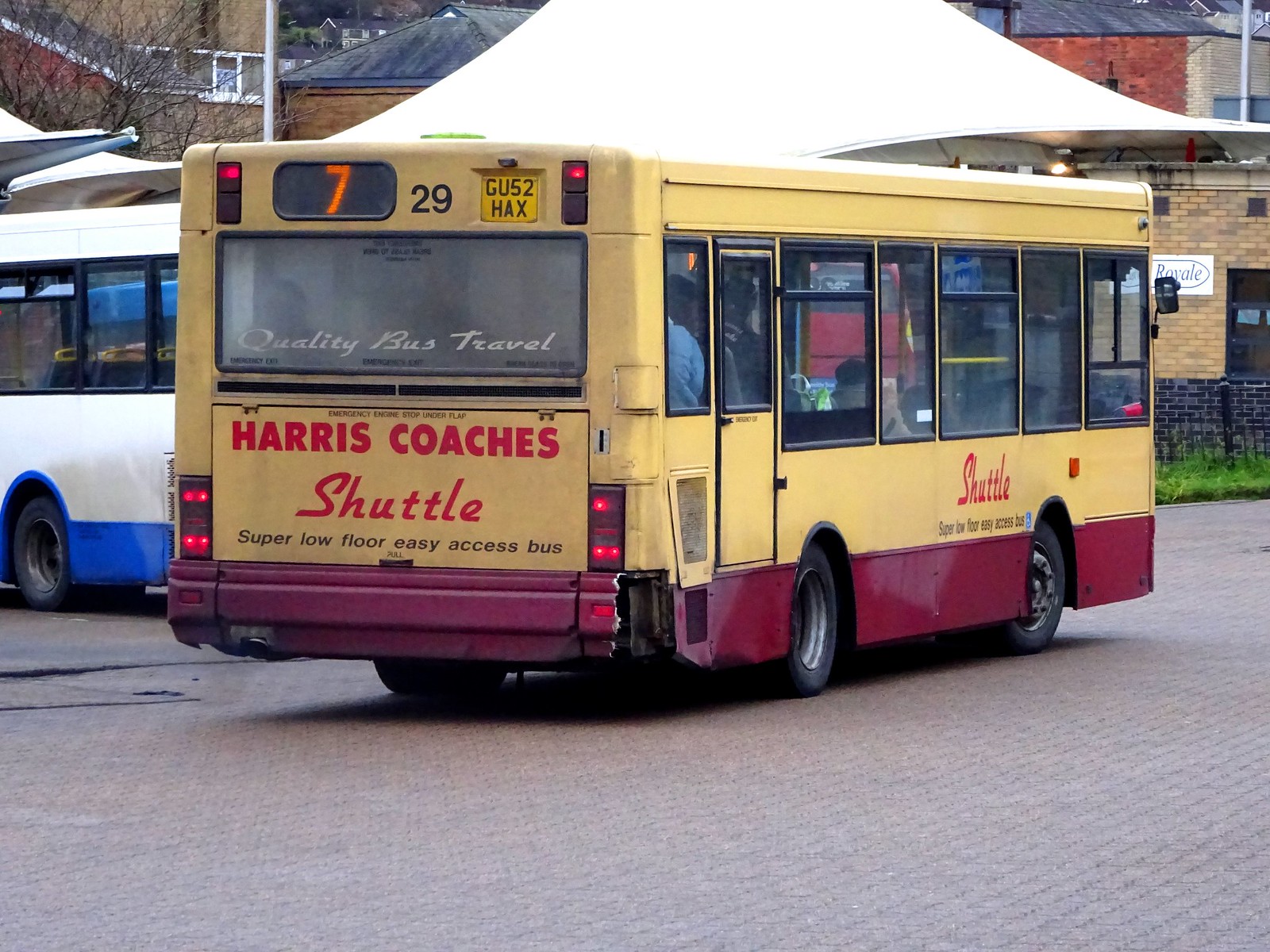This photograph features a distinctive, boxy yellow bus, prominently positioned on a grayish-black street with buildings in the background. This vehicle, identified as a Harris Coaches Shuttle, showcases its bright yellow body adorned with a red stripe along the bottom and a small section of purple near the tires and bumper. The back of the bus prominently displays "Harris Coaches Shuttle" in light red lettering and "Super Low Floor Easy Access Bus" just below it. Above these, the windshield features the slogan "Quality Bus Travel." At the top rear, a digital sign displays the number 7 and 29 alongside the license plate GU52HAX. Through the bus windows, a few passengers are visible. On the side, additional text reiterates "Shuttle Super Low Floor Easy Access Bus." To the left of this bus, a white bus with a blue stripe adds contrast to the scene. The overall setting suggests an urban environment with a brick-paved street.